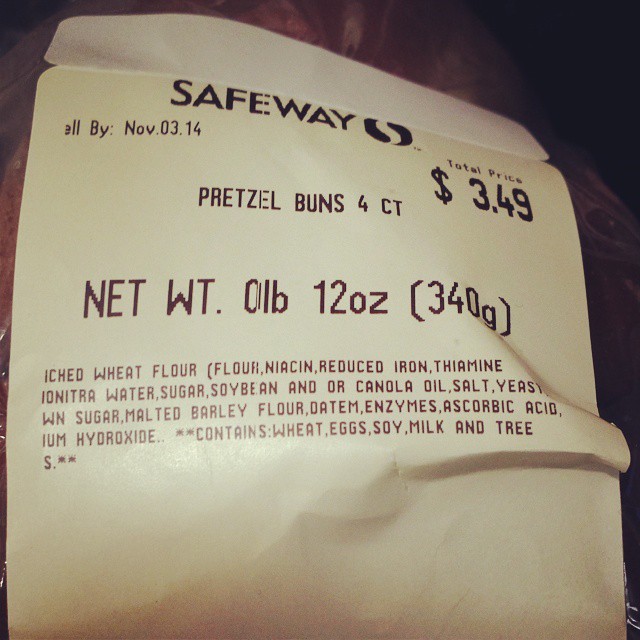This image displays a detailed receipt from Safeway. The receipt is printed on standard white paper with "Safeway" prominently featured in bold letters at the top. Directly underneath, the expiration date and batch number are listed as "L by November 03 14." 

The total price of the item is clearly stated as $3.49. The receipt details the purchase of pretzel buns, indicating "Pretzel Buns 4 CT" (where "4 CT" specifies a quantity of four buns). 

Below the product name is the net weight, expressed as "Net WT. 0 LB 12 OZ (340 G)" in parentheses, specifying the total weight of the buns.

The list of ingredients for the pretzel buns is thoroughly detailed as follows:
- Sweet flour (flour, niacin, reduced iron, thiamine mononitrate, riboflavin, folic acid)
- Water
- Sugar
- Soybean oil or canola oil
- Salt
- Yeast
- Diastatic malt (barley flour, malted barley flour)
- Enzymes
- Ascorbic acid
- Monocalcium phosphate
- Calcium propionate.

The ingredients note possible allergens, stating, "Contains: Wheat, Egg, Soy, Milk." 

The receipt adheres to formatting norms with standardized spacing and alignment, ensuring clarity of the printed information.